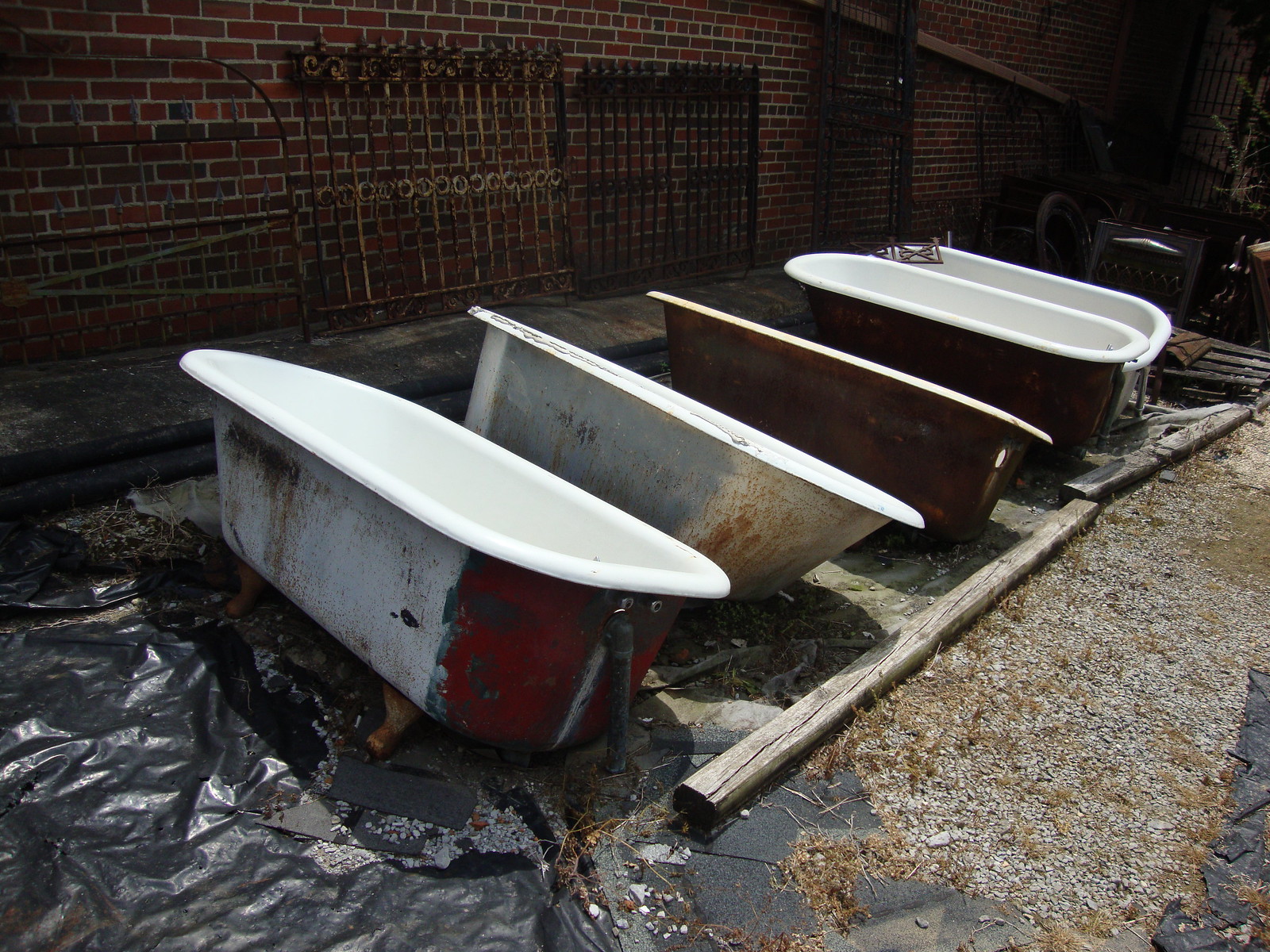In this daytime photograph, we see five old-fashioned, porcelain-style bathtubs with legs, arranged outdoors. The bathtubs are situated on a mix of gray, black, and discolored olive green tarps, suggesting exposure to weather. Their interiors are white, but their exteriors show signs of age, with varying degrees of rust and stains. The first bathtub has a white exterior with a red top, the second features a combination of white, dark gray, and rust-speckled white, and the third is chocolate brown with rust stains. The last two bathtubs are primarily white but also exhibit rust and aging.

The first three bathtubs lean to the right, with the third leaning so far that its interior is hidden, while the last two stand upright. In front of the bathtubs lie two wooden logs, similar to railroad ties, along with some brown leaves and gray to green gravel. The background displays a red, maroon, and black brick wall lined with decorative iron gates—one curved and two rectangular, with noticeable rust due to age. Behind the tubs are light brown railroad trusses, adding to the rustic, industrial atmosphere of the scene.